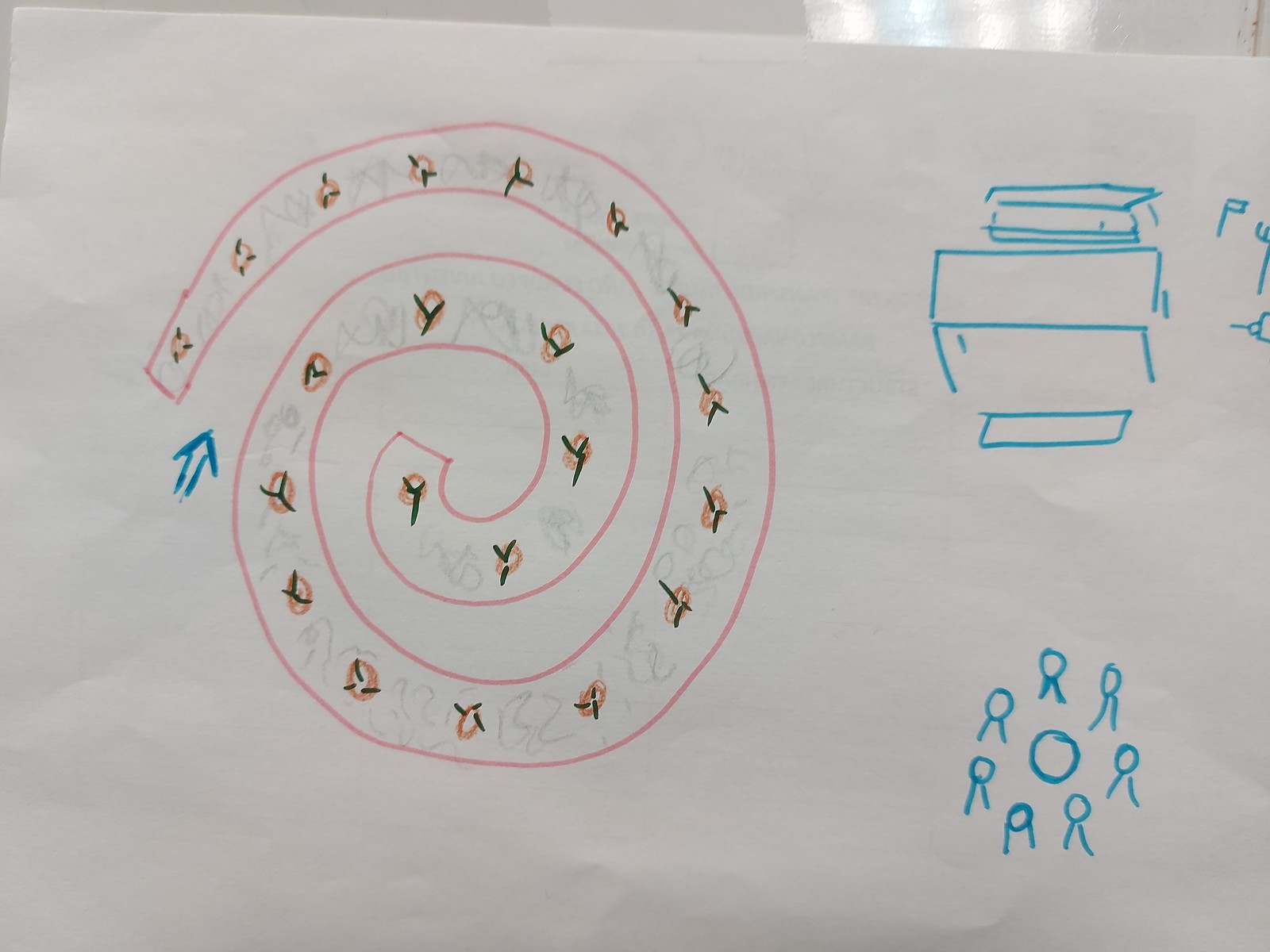In this photograph of a drawing on a plain white piece of printer paper, the captivating artwork is prominently displayed. On the right-hand side, delicate lines of a thin blue marker illustrate two distinct scenes. At the top, a long rectangular lunch table is depicted, complete with rectangular benches arranged along both its top and bottom sides. Below this, in the bottom right corner, a circular arrangement represents people seated around a table, with each figure portrayed using simple circles and lines to suggest shoulders or torsos.

Centrally positioned on the left, a large, elaborate spiral dominates the composition. This spiral, drawn and accentuated with a pink marker, is intricately detailed. Throughout the spiral, small orange circles are dispersed along the path, interspersed with grey squiggles penciled in to add depth and texture to the design. The contrast between the structured blue drawings and the fluid, colorful spiral creates a dynamic and visually engaging scene.